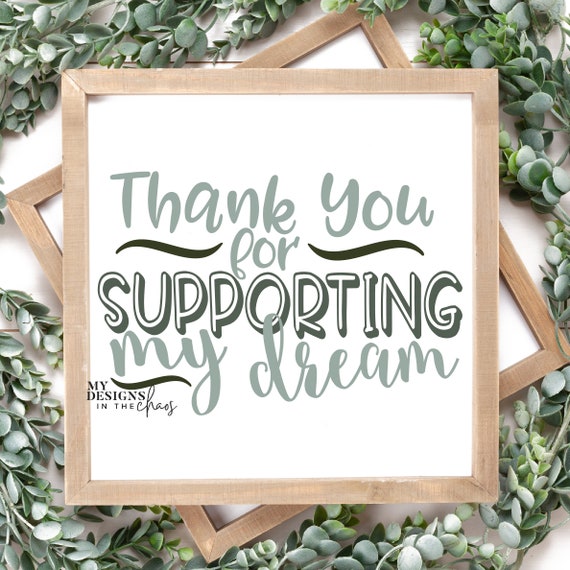The image shows a clear and well-lit photograph of a sign with a white background and borders of plain, uncoated light wood. The sign prominently displays the message "Thank you for supporting my dream" in green text, with some black elements and a squiggly line under the word "thank." In the bottom left corner, the sign reads "my designs in the chaos." This sign is placed at an angle on top of another similar sign, also featuring a white background and light wood frame. Surrounding the signs are decorative green leaves, enhancing the aesthetic appeal. The overall setting is bright, featuring a white background, possibly indicating the image was taken on a wall or a table.